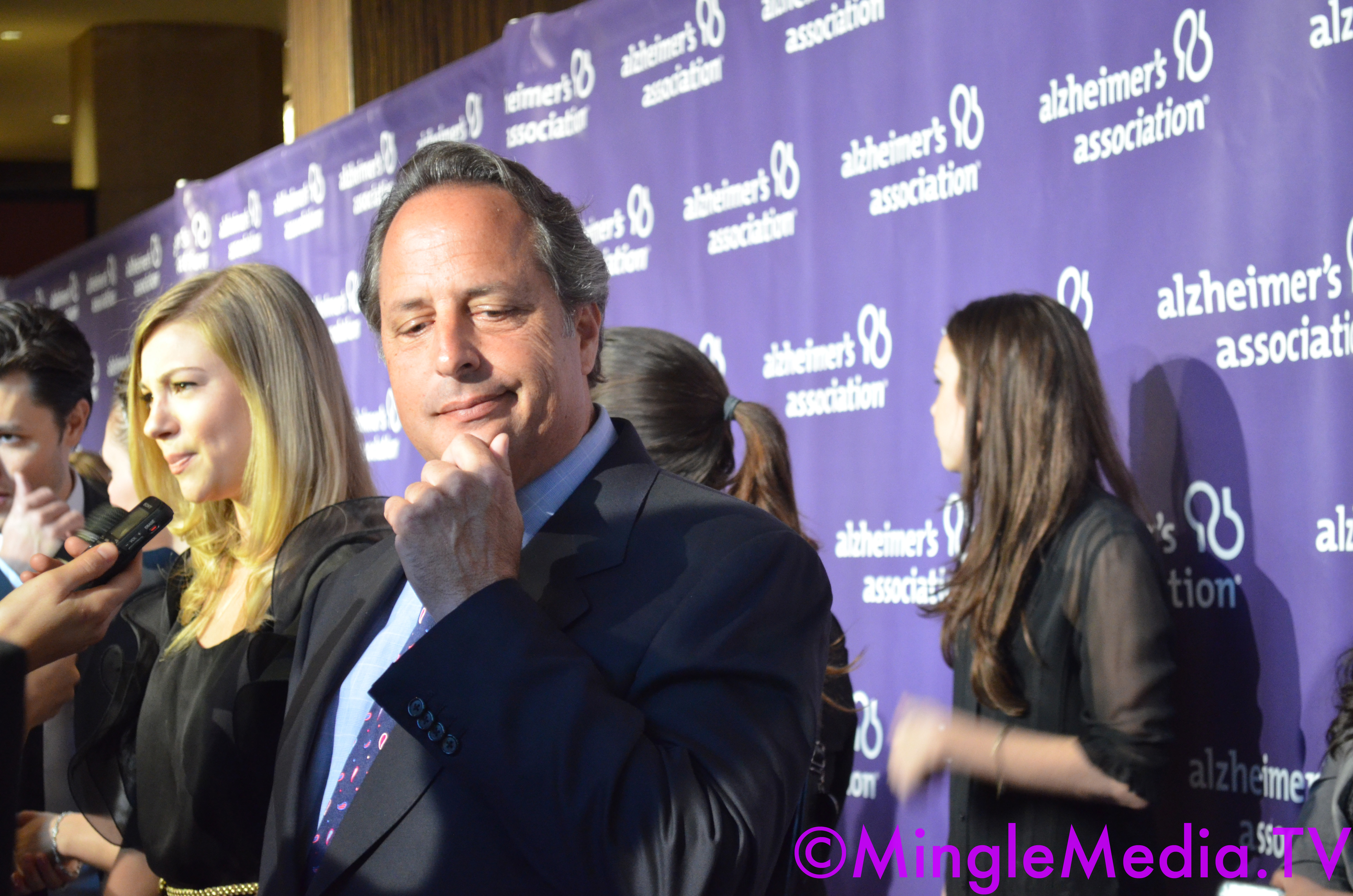The image depicts a lively scene at an Alzheimer's Association event, characterized by a star-studded red carpet atmosphere with attendees giving interviews and taking photographs. Prominently featured is a gentleman, likely John Lovett, with medium short-styled grayish hair, clad in a gray suit paired with a white shirt and a blue tie adorned with a jelly bean pattern. He strikes a contemplative pose, looking down with his left arm bent, hand held to his chin. To his right stands a blonde woman with long hair, engaged in conversation with someone holding a recorder. To his left is a dark-haired woman, her arm curving to the right as she likely converses with an unseen person. The backdrop is dominated by a blue banner repeatedly emblazoned with the Alzheimer's Association logo, providing a branded context to the event. The photograph, taken at a slight angle to the banner, captures the dynamic and bustling energy typical of high-profile premieres.